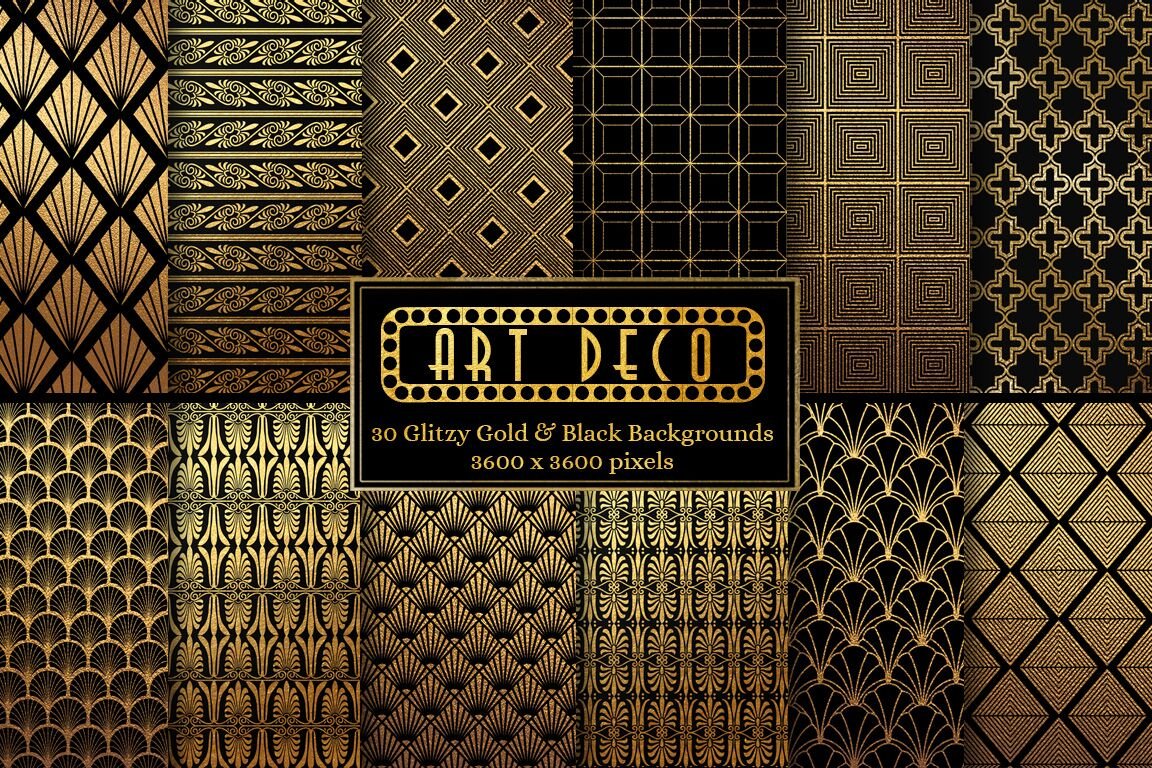This image features a central black rectangle bordered by a gold perforated oval frame, showcasing the text "Art Deco" in an elegant gold font. Below, it reads "30 glitzy gold and black backgrounds, 3600 by 3600 pixels." Surrounding this central focus are twelve distinct rectangular panels arranged in two rows of six, creating a landscape orientation. Each panel displays various intricate patterns of gold and black, including geometric designs, crisscross patterns, diamond shapes, floral motifs, and maze-like line work. The collection highlights the sophisticated and repetitive nature of these Art Deco-style backgrounds, all meticulously designed to exhibit opulence and elegance.